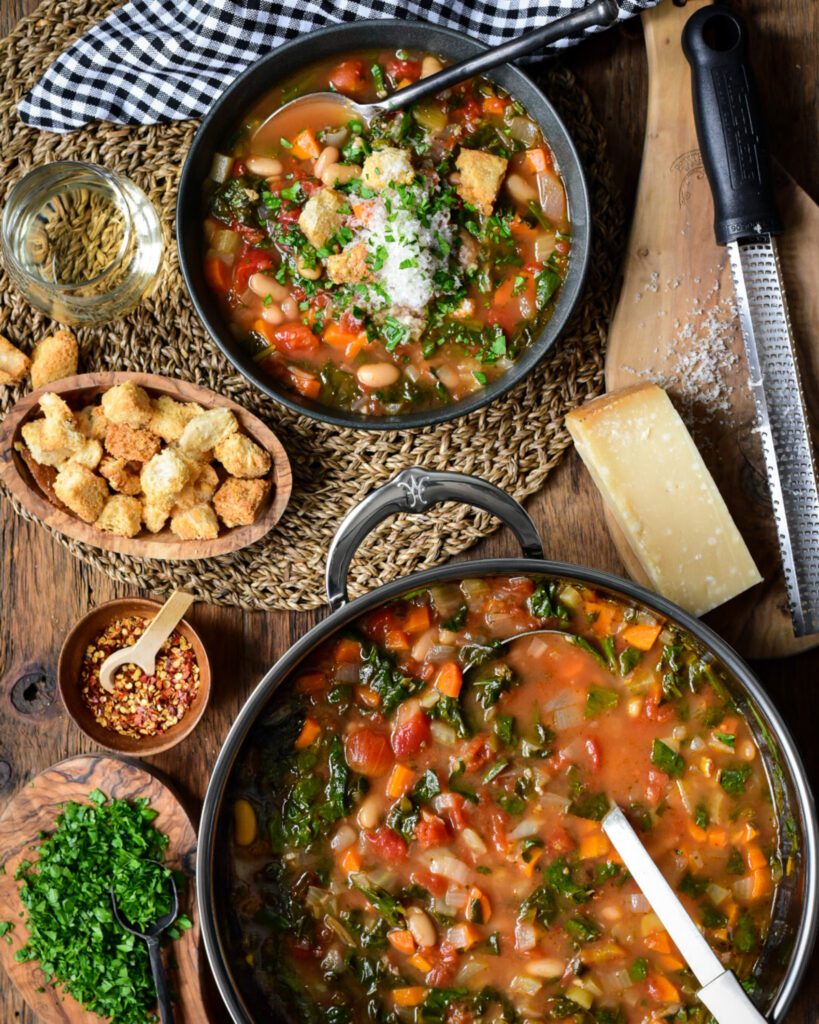The image is a detailed and vibrant aerial photograph of a dinner setting on a brown table laden with various food items. At the top left, there's a black and white Czech napkin placed on a brown pad. Adjacent to the napkin, a smaller bowl filled with a hearty soup is visible; the soup is topped with greens and Parmesan cheese, and a spoon is nestled inside the bowl. Next to the bowl, a glass with some liquid and a small wooden bowl full of croutons can be seen, suggesting a cozy and well-prepared meal setup.

The centerpiece of the image is a large, dark gray pot of vegetable soup located towards the lower right corner. This main pot of soup is rich and colorful, featuring ingredients like tomatoes, white beans, carrots, spinach, and possibly onions, all simmering in a robust tomato-based broth. A silver serving ladle protrudes from the pot, indicating that servings have been recently dished out. Between the large pot and the smaller bowl lies a small grater with a black handle, paired with a sturdy block of Parmesan cheese.

Completing the arrangement, there is a wooden cutting board with a brown spoon that holds fresh green herbs alongside another small wooden bowl containing additional herbs. This thoughtful dinner setting communicates warmth and attention to detail, offering a customizable dining experience where diners can add cheese, parsley, and other toppings to their preference.